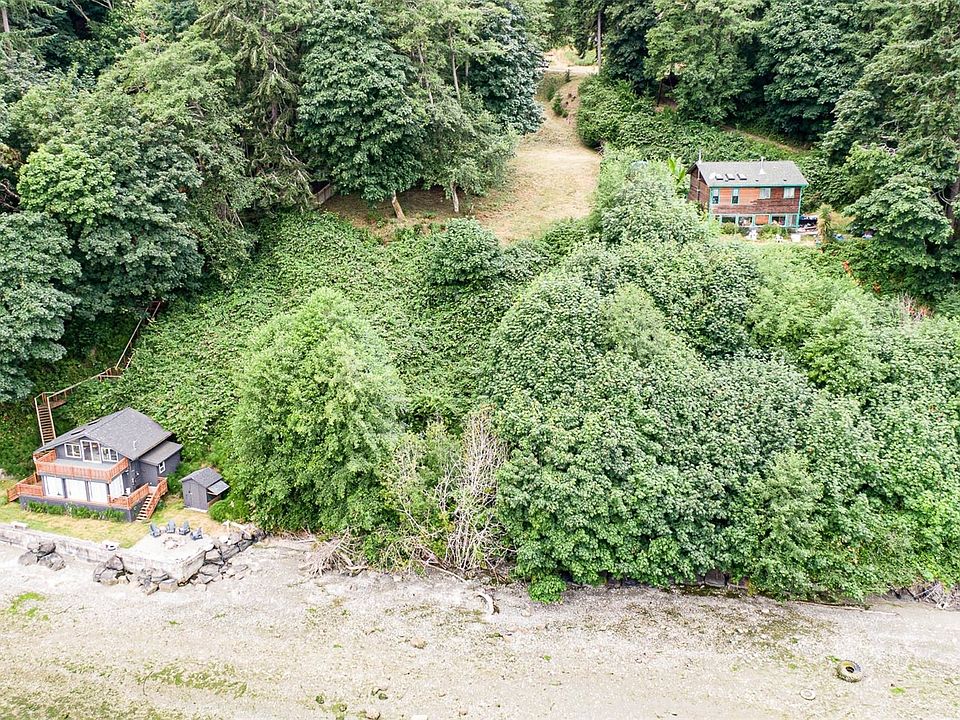This overhead image, likely captured using a drone or taken from a high vantage point, showcases a scenic, wooded landscape with two distinct houses nestled into the side of a lush green hill. The primary focus on the left-hand side is a large two-story gray house, featuring a gray roof, gray siding, and a wooden railing surrounding its deck. A prominent wooden staircase ascends from behind this house, climbing the hill and merging into the dense forest. On the right-hand side, another sizable two-story home stands out with its cedar-like wood siding, green trim, and a gray roof. Both houses are surrounded by an abundance of trees, indicating a heavily wooded area, with a gravel road visible at the bottom of the image providing access to this picturesque mountain setting.